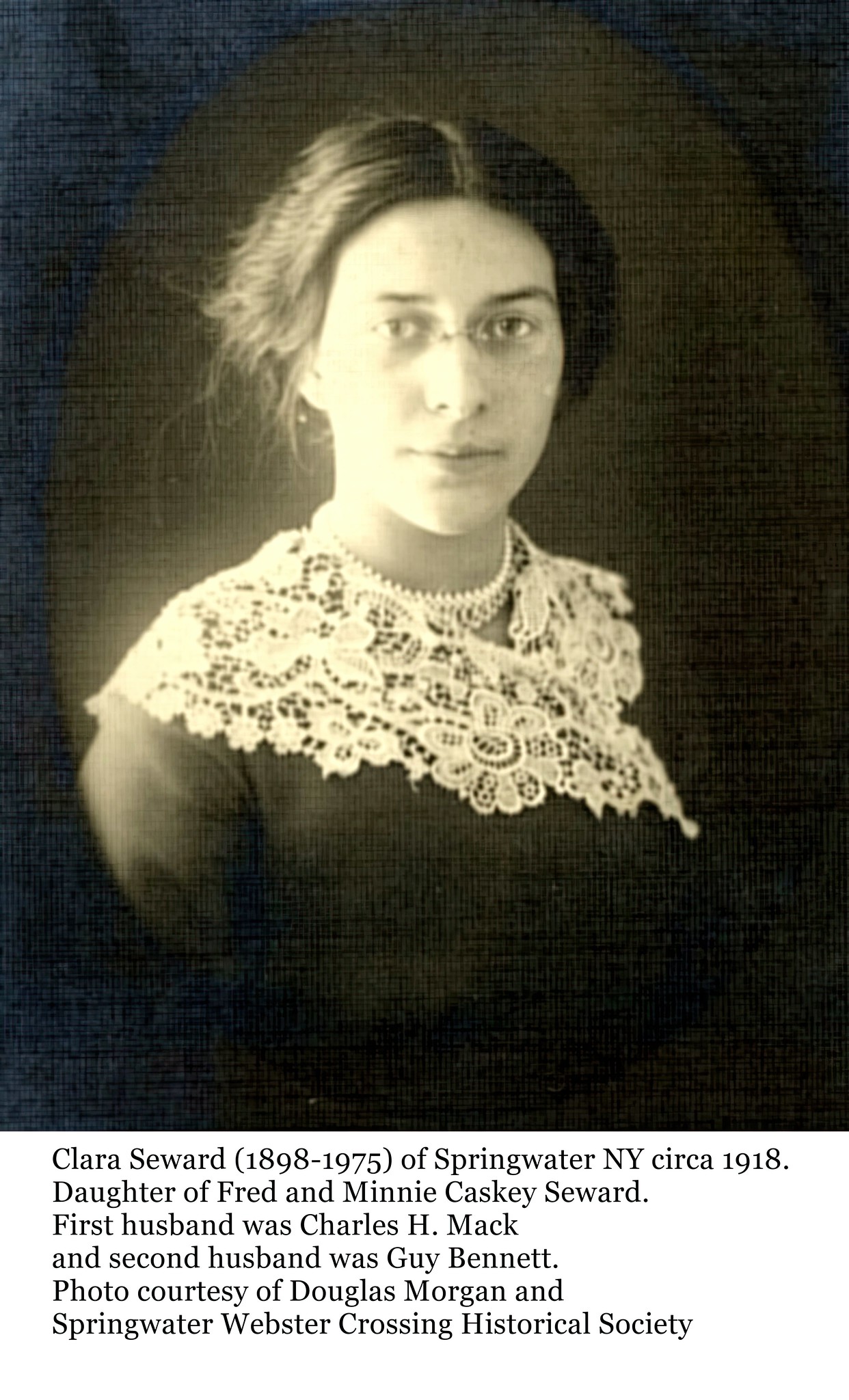The black-and-white photograph depicts Clara Seward, a young Caucasian woman, likely in her early 20s, taken around the year 1918. Clara, born in 1898 and passed away in 1975, hailed from Springwater, New York and was the daughter of Fred and Minnie Caskey Seward. In the portrait, Clara is adorned in a dark top featuring a delicate lace doily around her neck, resembling a shawl or elegant collar. She also sports a choker-style necklace and round, frameless glasses. Her dark hair is neatly parted down the center and pulled back. The photograph is courtesy of Douglas Morgan and the Springwater-Webster Crossing Historical Society, noting Clara's first marriage to Charles H. Mack followed by her second marriage to Guy Bennett.